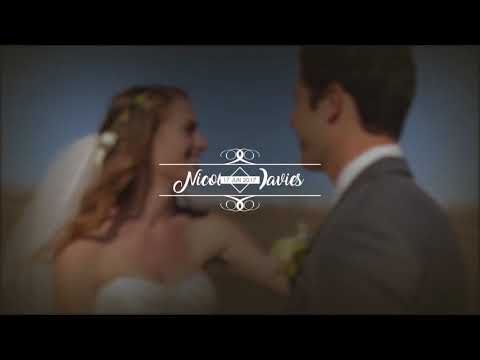This image appears to be a wedding photograph taken on June 17, 2017. It features a bride and groom against a bluish, slightly blurred background. The bride stands on the left side, facing sideways towards the right, and is joyfully smiling. She has long, wavy light brown hair, styled with a white veil or bridal headpiece attached at the back. Her strapless white dress, likely with a sweetheart neckline, suggests elegance. The groom stands on the right, turned at a three-quarter angle with his face mostly obscured. He has short dark hair and is dressed in a gray suit complemented by a white undershirt and a corsage on his lapel. Despite the overall blurriness and faded quality of the image, the joy and significance of the moment are palpable. The text "Nicole Davies" is visible, marking the occasion and providing a personal touch to the cherished memory.